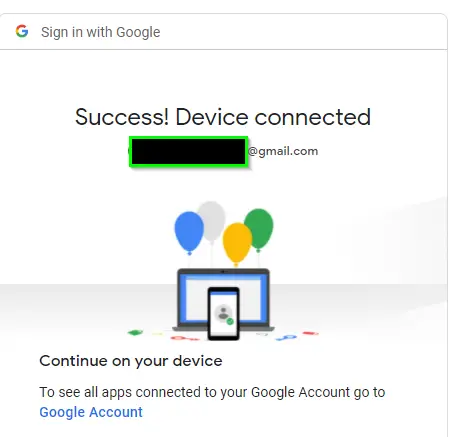This image is a screenshot of a Google account confirmation page. The top of the page features a Google banner with a noticeable "Sign in with Google" button, alongside the recognizable but simplified "G" Google logo. Centrally displayed on the page, there is a prominent black text message reading "Success! Device connected," followed by a specific Gmail address, which seems to be the email associated with the connected device.

Beneath this message, there is an illustrative graphic that includes a laptop with a smartphone positioned in front of it. Above these devices, there are four balloons in varying colors—blue, gray, yellow, and green—adding a celebratory touch to the confirmation.

Around the laptop and smartphone graphic, there are several key icons. These icons likely symbolize that the devices and account are secure and have been successfully linked. Below the graphic, there is a directive text encouraging the user to "Continue on your device." An additional note at the bottom advises users to visit their Google account settings to see all apps connected to their account.